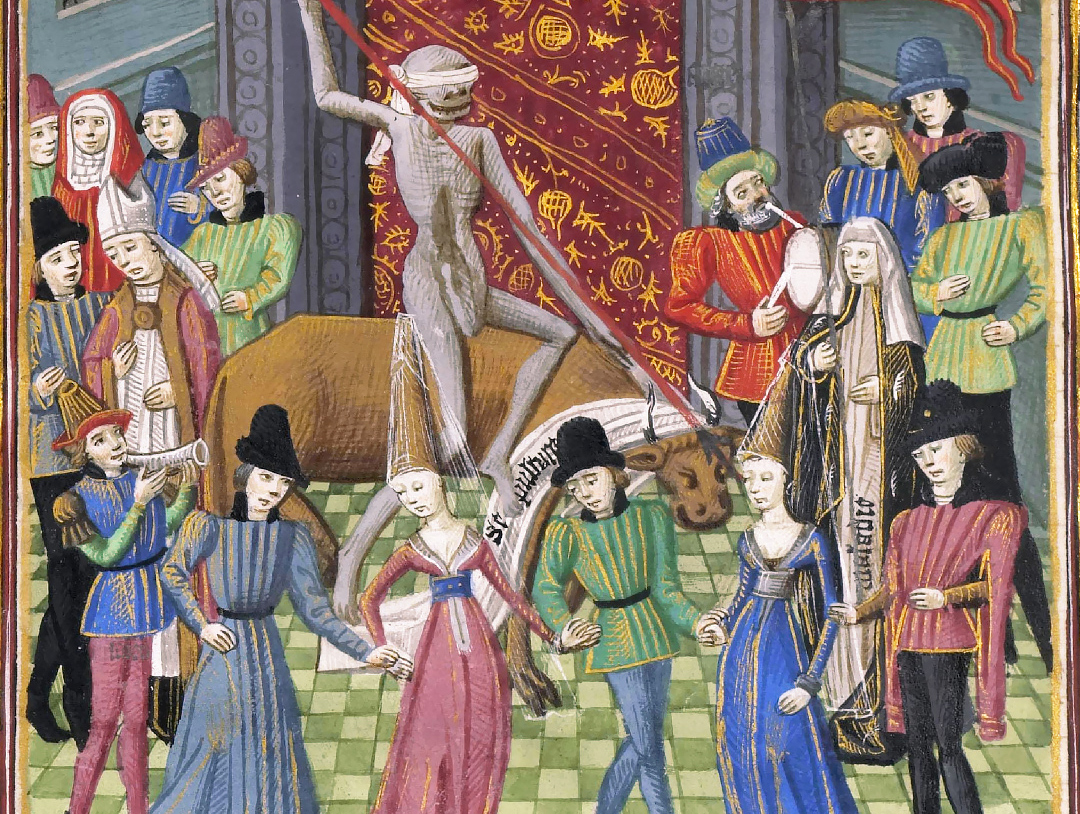The painting "Dancing Mania" by Pierre Mikoltz, possibly reflecting themes from the Middle Ages or the Black Death of 1348, unfolds in a green and white checkered floored room with grayish-blue walls. At the center stands a skeletal, mummy-like figure, blindfolded, and holding a long, angled red spear. This figure ominously looms in front of what could be an oxen or buffalo and is backed by a large red and gold tapestry. On either side and at the bottom, groups of men and women, appearing somber and melancholic, are dressed in pink, blue, and green dresses, some accessorized with black top hats and lacy, pointed veils. Among these figures, to the right of the spear's point, stands a young lady in a blue dress with a maiden’s hat, drawing particular attention. Some noblemen in purple, green, and blue attire are also present, one being a court jester. A composition full of detail and melancholy, this intricate scene is accentuated by its vivid and rich colors.